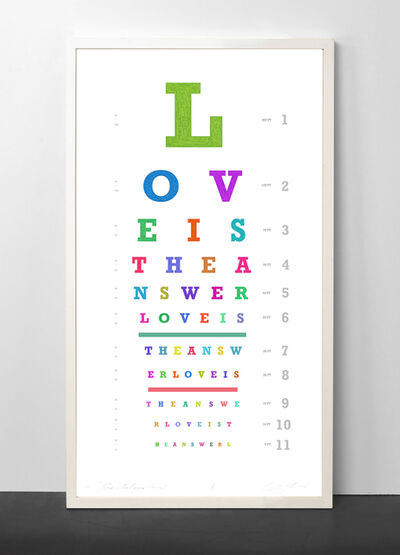The image displays a stylized novelty eye chart mounted in a white frame against a white wall with a grey surface beneath it. This decorative eye chart features the repeated phrase "Love is the answer," with the letters decreasing in size as they descend down the chart, mimicking a traditional eye test format. At the top, there is a prominent lime green letter "L," followed by slightly smaller blue "O" and purple "V" letters. Below this, the letters "E," "I," and "S" appear in green, red, and turquoise colors respectively. The pattern continues with the letters "T," "H," "E," "A," "N," "S," "W," and "E" in varying shades of pink, blue, brown, yellow, and purple. The sequence repeats with similar color variations, each line smaller than the one above, creating a colorful and diminishing visual narrative. The eye chart is also marked by numbers 1 through 11 in light gray on the far right, emphasizing the eye test motif. The vibrant and multi-colored letters convey the recurring and positive message "Love is the answer" throughout the entire chart.